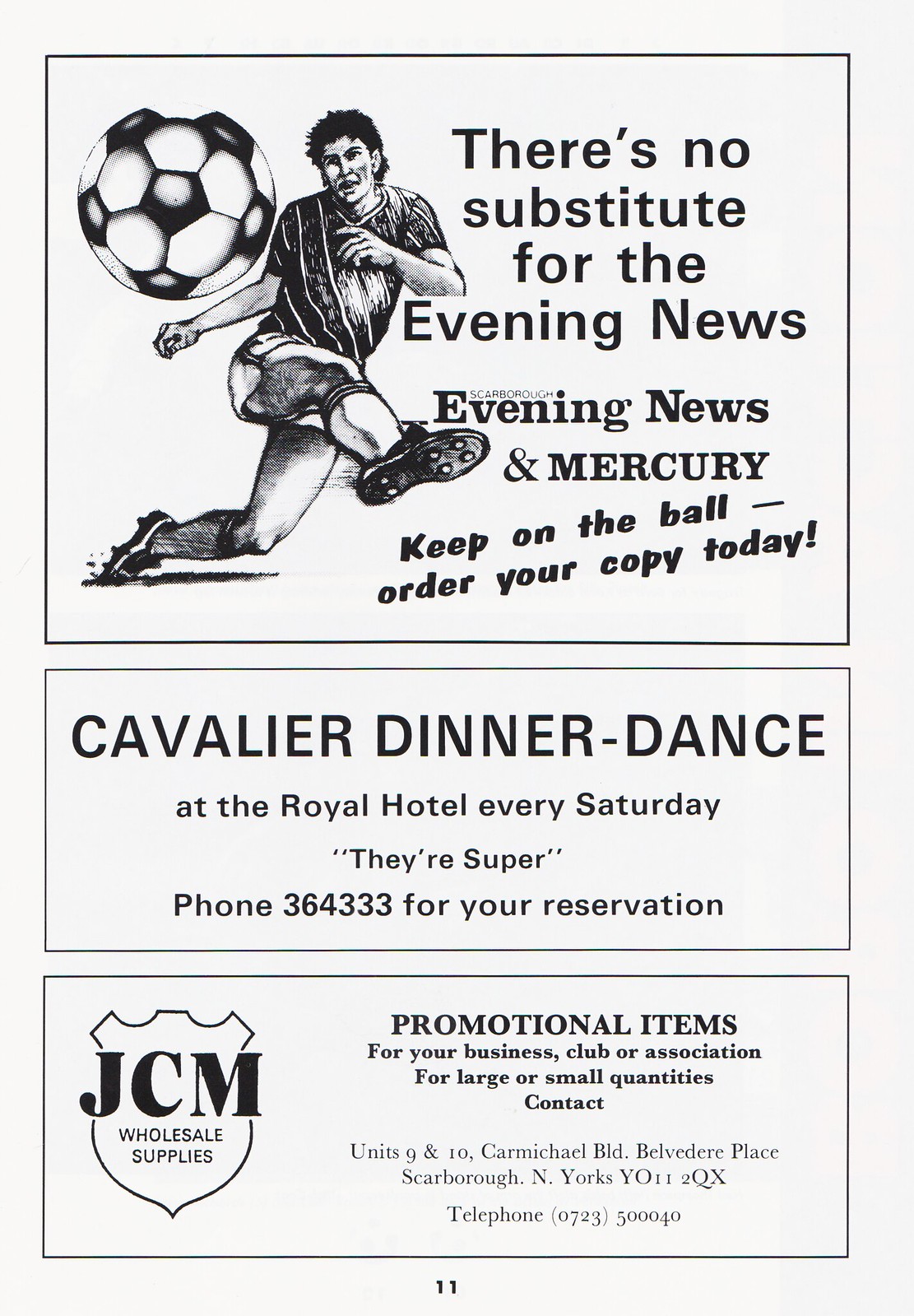The vertically aligned rectangular image appears to be a black-and-white page from an old magazine featuring three distinct advertisements, each enclosed in thin black borders. At the top, the most prominent ad showcases a hand-drawn illustration of a soccer player kicking a large soccer ball positioned in the upper left corner. Adjacent to the drawing, the text reads in serif and sans-serif fonts, "There's no substitute for the evening news." Below, in a custom handwritten font, it continues with, "Evening News and Mercury. Keep on the ball. Order your copy today."

The middle section contains the second advertisement for the "Cavalier Dinner Dance." The text, presented in all capital letters, announces, "At the Royal Hotel every Saturday." The phrase "They're super" is highlighted in quotes, followed by a reservation phone number: "Phone 364-333."

At the bottom, the third advertisement is dedicated to "JCM Wholesale Supplies," whose logo appears on the left. The bold text promotes, "Promotional items for your business, club, or association." Below that, it details, "For large or small quantities, contact Units 9 and 10 Carmichael Boulevard, Belvedere Place, Scarborough, New York Y0112QX." Lastly, the ad provides a contact telephone number: "0723500040." In the center at the bottom of the page, the page number "11" is visible.